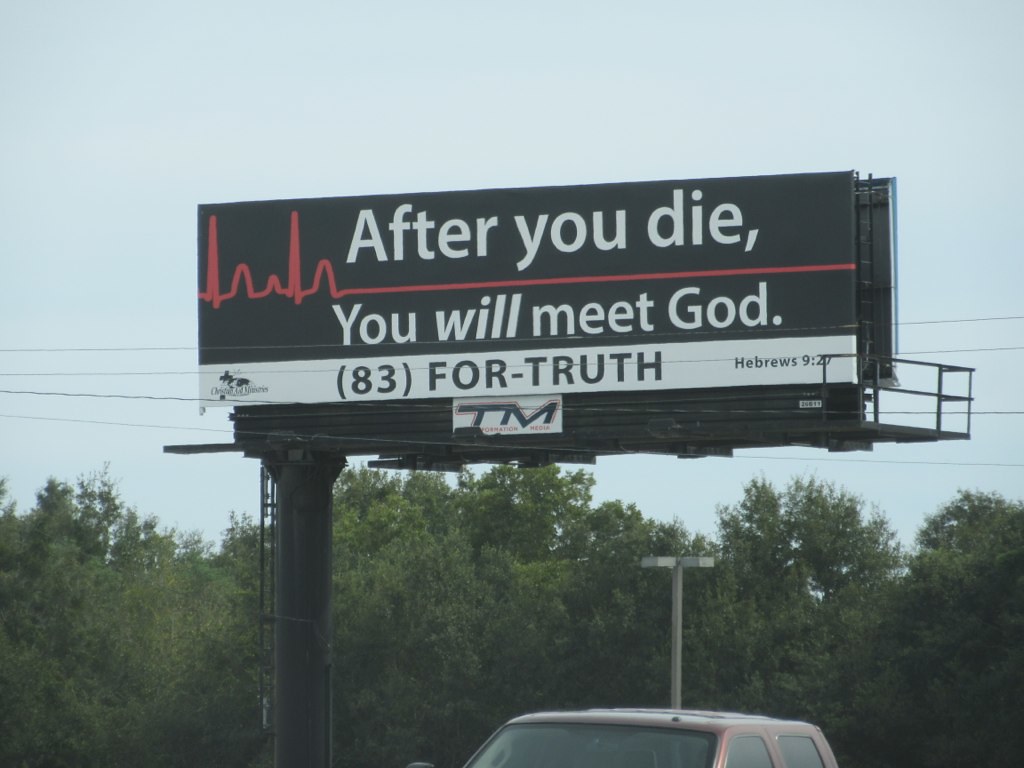This detailed real-life photograph captures a striking billboard as its central focus. Dominating the image, the billboard displays a poignant message in bold white text: "After you die, you will meet God." Between these lines of text, a red electrocardiogram-style line, reminiscent of a hospital monitor's lifeline, underscores the gravity of the message. The billboard's background is stark black, with a white bar across the bottom containing text in black: "(83) 4-TRUTH" followed by "Hebrews 9:20" in smaller letters.

The billboard structure itself is supported by a thick metal pole, and the branding "T and M" is visible, possibly indicating the advertising company. Cutting across the image are several electrical and telephone lines, which add a layer of urban detail.

The sky behind the billboard is overcast, painted in a light blue hue that suggests a cloudy day, despite the absence of visible clouds. The background is filled with the tops of lush, bushy green trees, creating a natural wall of greenery.

In the lower center of the image, the dark red top of an SUV or truck is partially visible, heading towards the viewer, with its windshield and side windows clearly shown. Behind this vehicle, a streetlight stands tall, adding to the urban landscape.